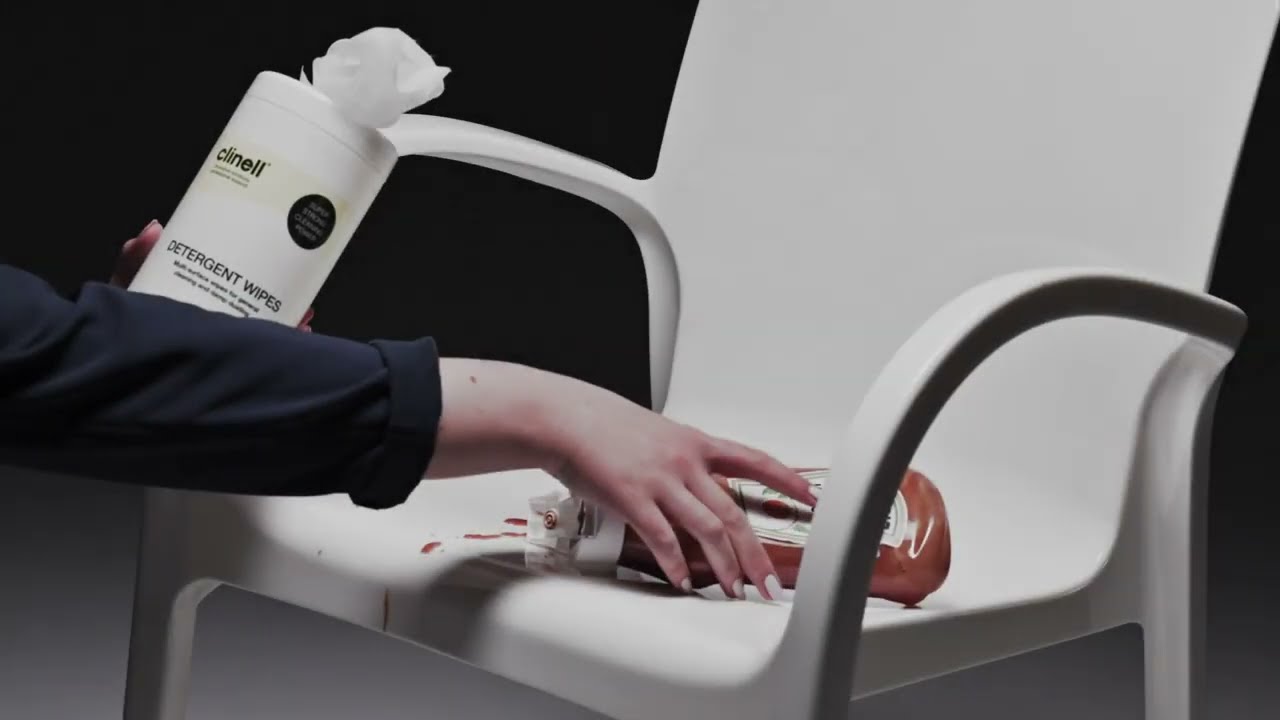The image portrays a meticulously staged scene, likely an advertisement, showcasing a woman cleaning a ketchup spill on a white plastic chair. Her arms, clothed in a black shirt with sleeves rolled up, extend from the left side of the image. The woman’s right hand, with white-painted fingernails, reaches forward to grasp an open red ketchup bottle lying on its side on the chair seat, which has created a mess of smeared ketchup. Her left hand strategically holds a container of CLINELL detergent wipes, positioned so the logo is clearly visible to the camera. The scene is set against a gradient gray background, dark at the top and transitioning to light gray at the bottom, emphasizing the cleaning action and the product. This detailed depiction captures the poised moment before she cleans up the spill, illustrating both urgency and readiness.